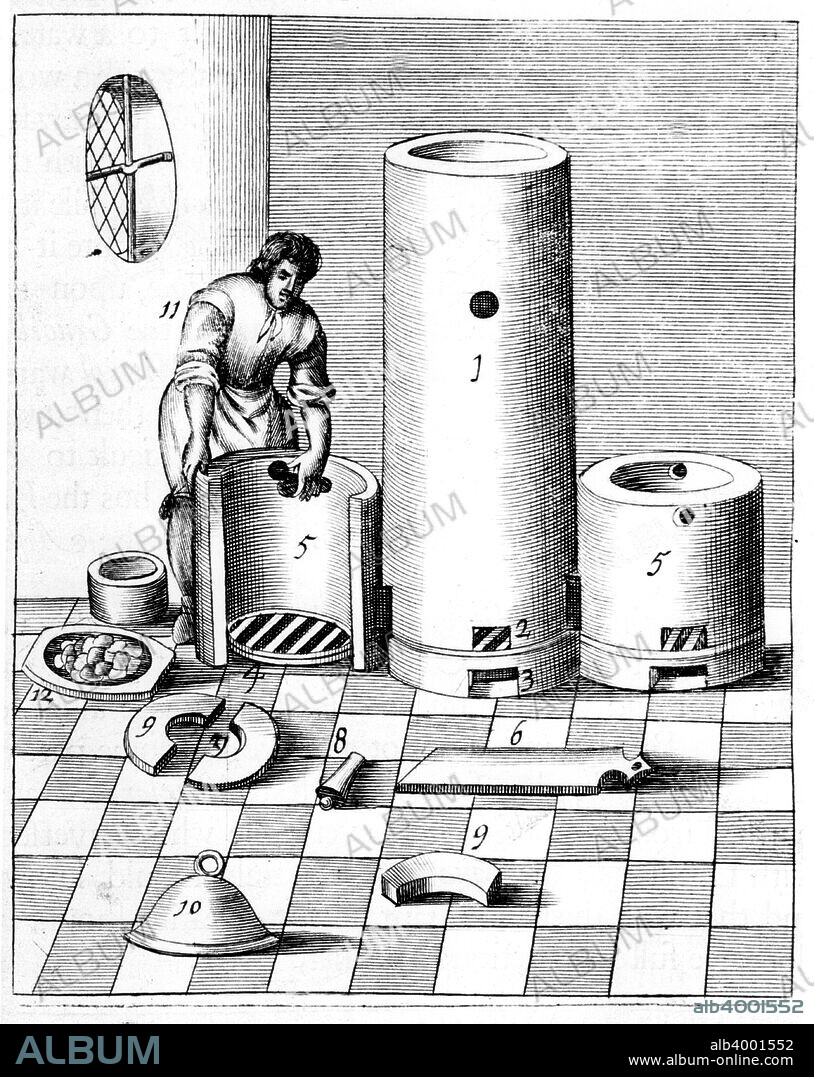This black-and-white drawing captures a meticulous scene where a person is engaged in constructing or assembling an object using various numbered pieces scattered on the ground. The person is positioned in front of three cylindrical structures; two of these structures are of the same height, approximately reaching the person's thigh, while the third, taller cylinder stands between them, towering over the individual. One of the cylinders is open, and the person is seen placing an item inside it, suggesting an ongoing process or task. 

The backdrop features a window, adding context to the setting, possibly an indoor environment such as a workshop or laboratory. Intriguingly, each piece on the ground bears a distinct number (1, 6, 9, 8, 9, 10, 12), hinting at an organized, step-by-step assembly process.

The image is marked with a prominent gray watermark, diagonally reading "ALBUM" in capital letters across its entirety. Along the bottom, a solid black strip runs horizontally, bearing the word "ALBUM" also in capital letters. On the far-right end of this strip, the website "www.album-online.com" is printed in a clean, white font, offering a source or reference for the image.

This detailed depiction is rich with elements of focus, structure, and an air of methodical creation, visually engaging viewers with its intricate details and composition.